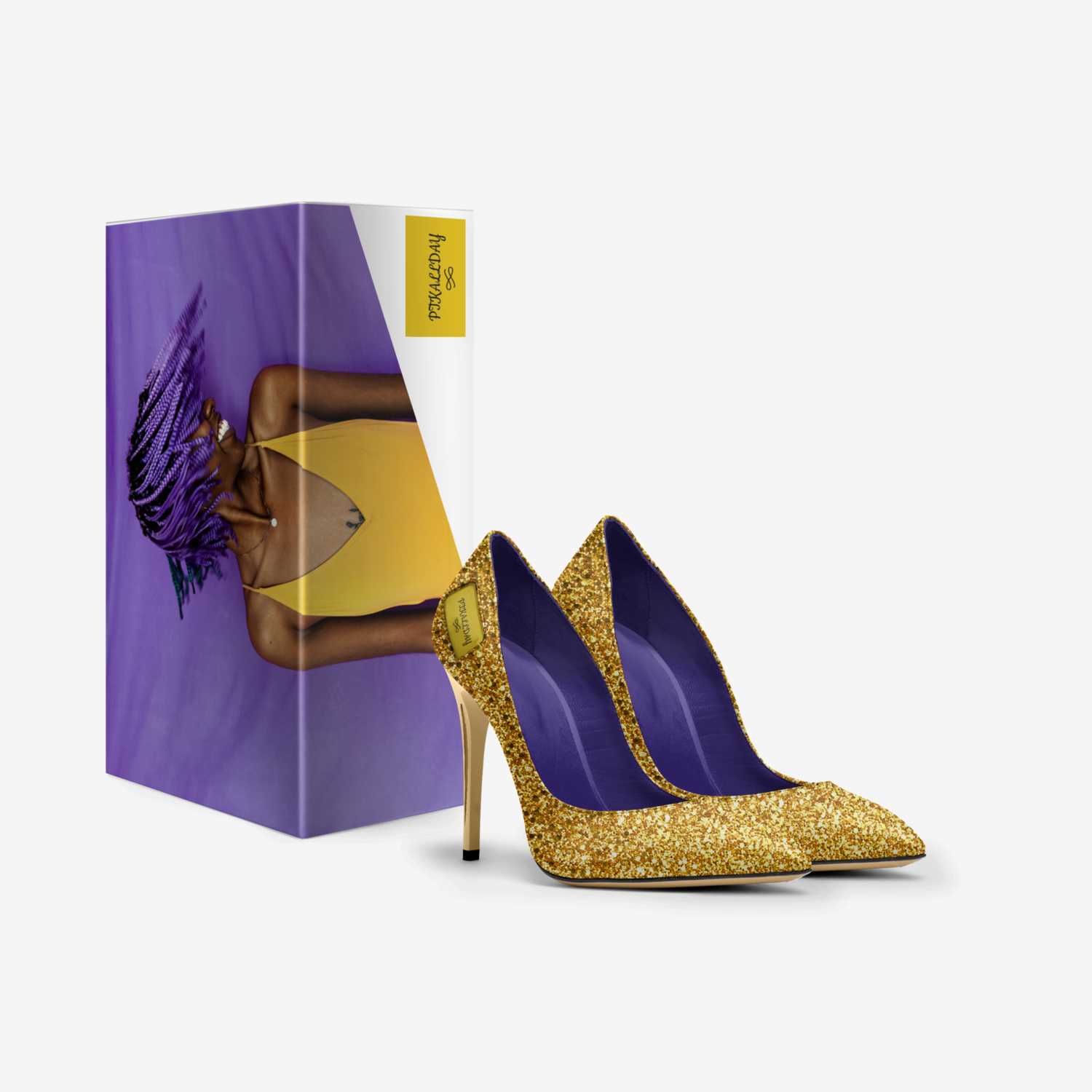The image showcases a pair of high-heeled shoes with a dazzling diamond-like glittery exterior, giving them a goldish shimmer. The heel is smooth gold with a black rubber tip. The inner lining of the shoes is a deep royal purple, featuring a gold label or patch on the back. Beside the shoes, there is a shoe box decorated with an image of a dark-skinned woman with purple braided hair, wearing a yellow tank top. The woman stands against a purple backdrop. The shoe box is primarily purple and white and bears a small, somewhat illegible yellow text box located at the top right corner. Both the shoes and the box are set against a clean white background, making the glitter and colors stand out vividly.